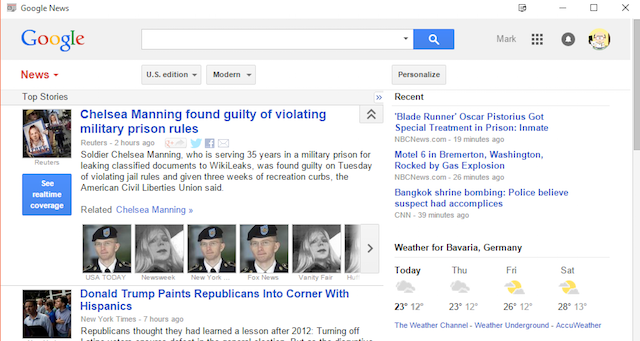This image is a detailed screenshot of a Google News webpage, presented in a left-to-right horizontal format. The white background, characteristic of many web pages, is interrupted on the left side by a thin red vertical line. On the right side, there is a visible scrollbar, framing the content. The top and bottom borders of the image are unmarked, providing a seamless view.

In the upper left corner, the "Google News" header is prominently displayed alongside icons that offer various functionalities (likely related to settings and profiles). To the right of these icons, the traditional set of window control buttons (minimize, maximize, and close) are visible, positioned in the upper-right corner of the screen.

Below this header section, a gray bar stretches horizontally across the image. This bar features the renowned Google search bar, complete with the blue-background magnifying glass icon, which is white. Adjacent to the search bar is "Google" in its colorful typographic logo. Alongside, there are additional icons including a profile picture icon that users can click on for more options. The word "News" is highlighted in red, indicating the current section being viewed.

The main content area of the image shows the US Edition of Google News, tailored and personalized for the user. The top stories are prominently displayed with headings such as "Chelsea Manning found guilty of violating military prison rules," providing readers with pertinent details about the news. Another highlighted story covers "Donald Trump paints Republicans into a corner with Hispanics," again followed by additional information.

On the right side of the main content, there's a section titled "Recent," showcasing the latest articles, their sources, and timestamps indicating how recently they were published. Below this, there's a localized weather update for Bavaria, Germany, including a three-day forecast from Thursday through Saturday.

This screenshot comprehensively illustrates the layout and elements typical of a Google News webpage, offering insight into its structure and the type of content one might encounter there.